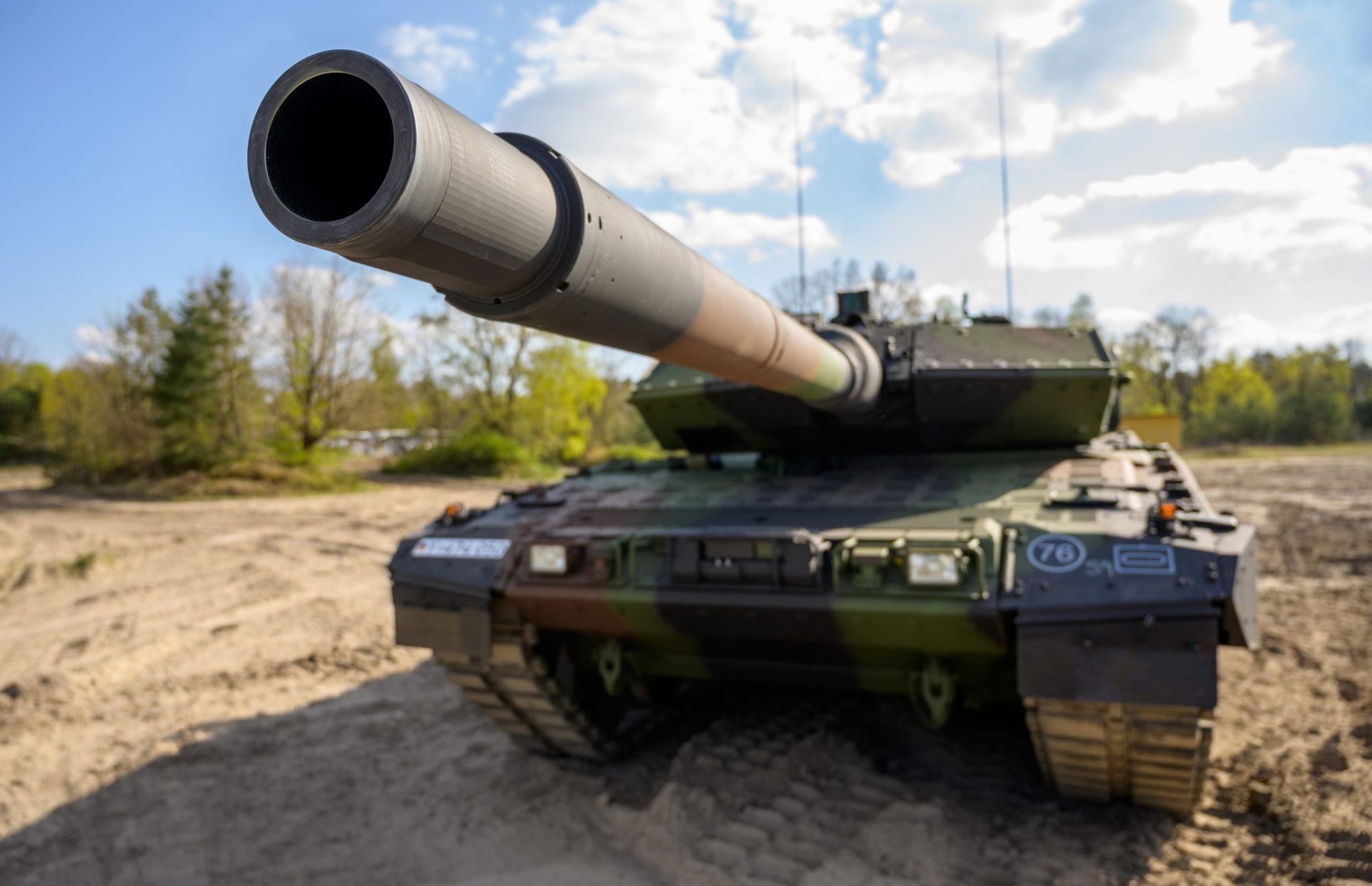This daytime photograph captures a military tank positioned in a dirt field heavily marked by tire tracks. The tank, adorned in a green, brown, and black camouflage pattern, features prominent white lettering "76" and a white circle on its front. It’s equipped with a large cannon extending from its main body, aimed slightly to the left in the frame. The tank also has large rubber tracks and is likely fitted with two black antenna masts. The scene is set against a line of sparse trees, under a partly cloudy sky with a visible sun flare. The overall setting suggests ample open space for the tank's maneuvering.